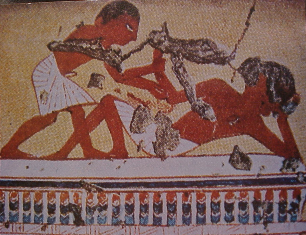The image features a close-up of an ancient Egyptian painting, likely from a tomb or monument, depicting two men with dark brown to reddish-brown skin engaged in an interaction. One man is reclining on a decorated platform, his head resting in his hand, while the other man stands above him. The standing man appears to be reaching out, possibly to help the reclining man up, suggesting a gesture of assistance. Both men are dressed in traditional white loincloth skirts. The platform they are on is adorned with intricate red, blue, and white mosaic patterns and supported by white columns, with a sand-colored background above it. The painting shows signs of aging and damage, with some elements and details obscured or distorted.